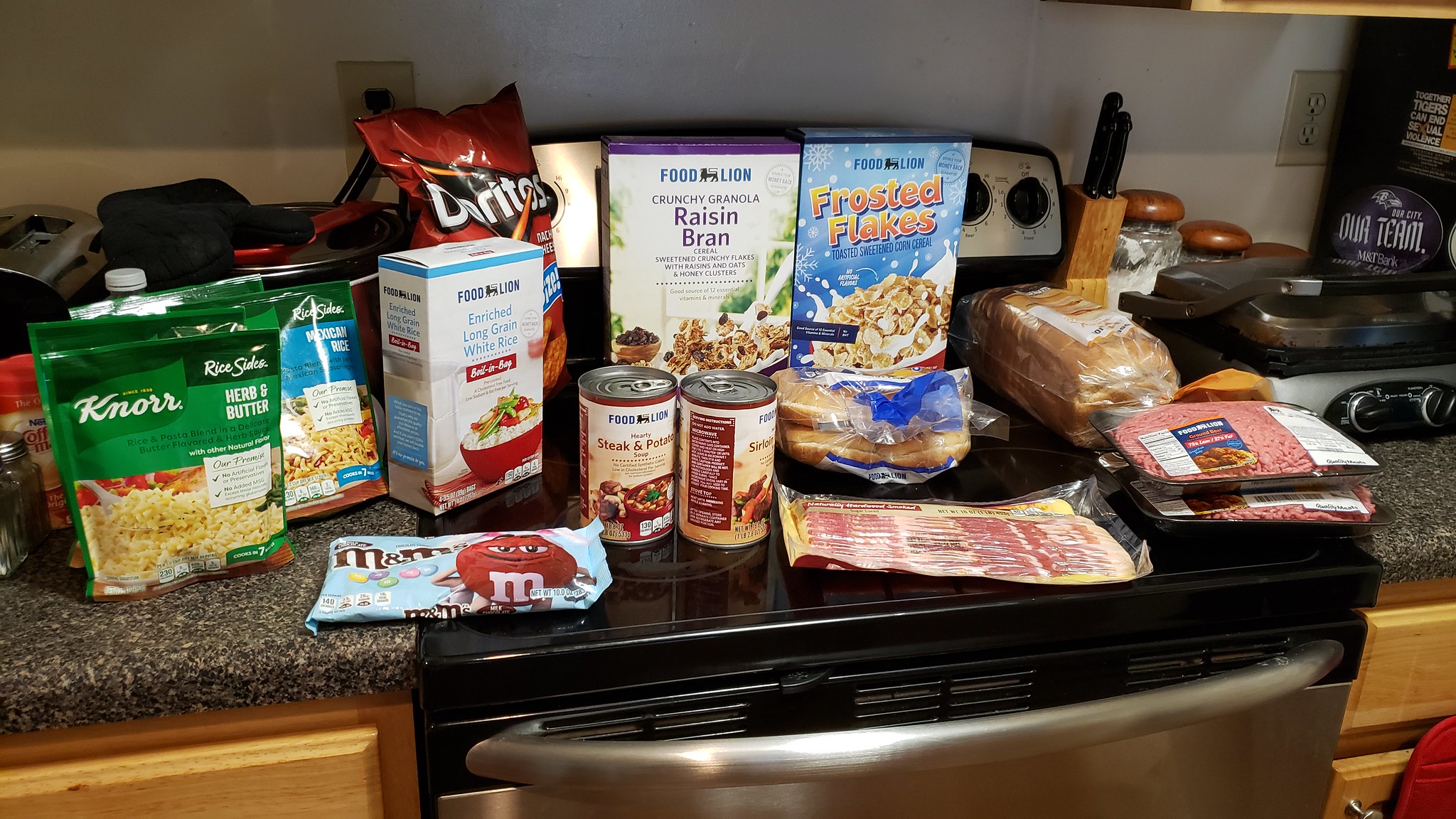This photograph captures the interior of a well-lit kitchen with counters laden with an array of grocery items. The centerpiece is a modern stove with a sleek black induction cooktop and a stainless steel oven, partially visible, with its handle prominently in focus. Flanking the stove are dark gray granite countertops that stretch out to either side, providing ample space for the displayed items. The kitchen cabinetry below is made of light blonde wood, contributing to a warm, natural ambiance.

On the stovetop and counters, a variety of food products are meticulously arranged. Among them are two packages of ground beef, a sealed yellow package of bacon, and several types of rice, including a green Knorr herb and butter rice and a box of enriched long-grain white rice. A vibrant bag of pastel-colored M&Ms and a large bag of Doritos stand out against the countertop. Additionally, there are two large cans of steak and potato soup, a loaf of bread, and a package of hamburger buns, all neatly placed. Breakfast cereals such as Raisin Bran and Frosted Flakes add to the assortment.

To the left of the stove, an electrical outlet is occupied, while the one on the right is empty. A knife block with two knives is positioned to the stove's immediate right. The kitchen scene is completed with hints of additional wood-paneled drawers beneath the counter, suggesting a clean, organized environment even amidst the grocery display.